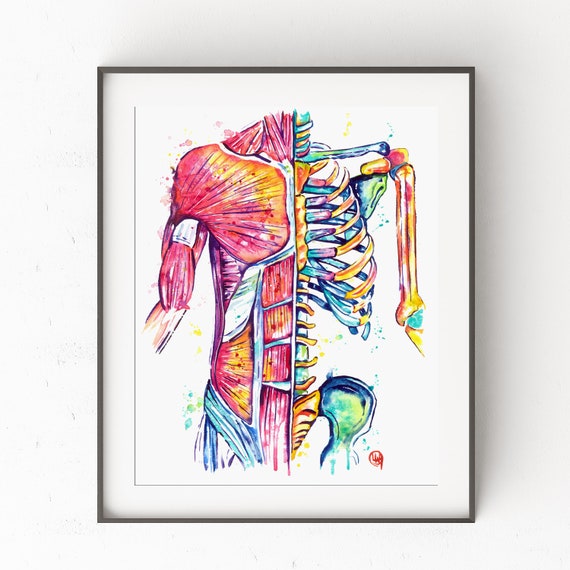This detailed artwork is a painted depiction of the human body, artistically captured in a black-bordered frame with a white backdrop. The frame features a distinctive black L-shaped line running from the top left to the bottom right. The painting vividly presents a bifurcated view of the human form, dividing it vertically down the center. The left side of the image vividly showcases the muscular structure, where muscles and tendons are rendered in vibrant colors of pink, orange, blue, and green. The right side reveals the skeleton, highlighted with hues of yellow, purple, blue, green, gold, and pink. Seen from the neck down to the pelvis, the painting includes detailed renderings of the arms and a glimpse of the legs. The artwork contrasts the anatomical intricacies of muscles and tendons against the stark, detailed bones of the skeleton. Additionally, there appears to be a red, squiggly signature within a circle at the bottom, though it is not legible. The painting beautifully merges art and anatomy, showcasing a striking comparison between the internal structures of the human body.